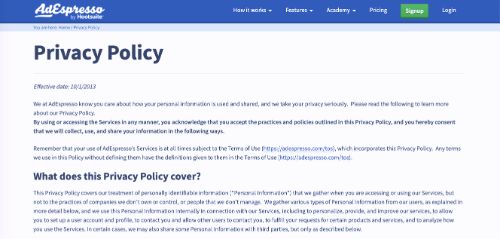Screenshot of the AdEspresso Website - Privacy Policy Page:

The screenshot showcases the AdEspresso website, identifiable by its name displayed prominently in the top left-hand corner in a white cursive font against a blue background. The top portion, featuring the website name, transitions into a white background with blue text. To the right of the website name, a navigation menu contains six categories: "How It Works," "Features," "Academy," "Pricing," a green button with white text labeled "Sign Up," and a "Log In" link.

Below this top navigation, a light blue banner spans the width of the webpage, but the text within it is difficult to discern due to blurriness. The primary content of the displayed page focuses on AdEspresso's Privacy Policy. While the effective date is visible, it remains unreadable because of the blur. The policy details commence with an introduction and a section titled "What Does This Privacy Policy Cover?" Several terms and conditions are interspersed with highlighted blue links, which presumably direct users to the website’s Terms of Use and other relevant documents, allowing users to examine them before agreeing to the privacy policy.